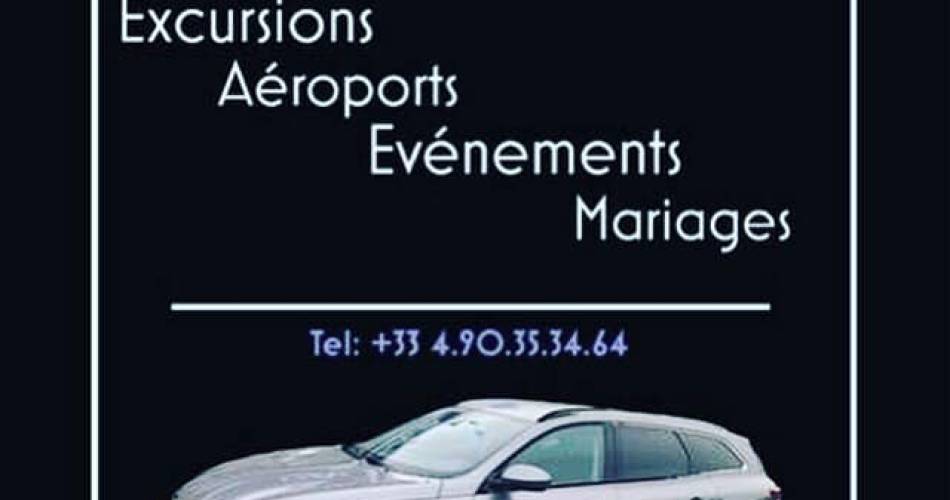The image features a modern, silver station wagon illuminated by natural daylight on a black background. On either side of the image are vertical white stripes positioned a bit inward from the edges. At the top of the image, the words "Excursions" appear on the left, followed by "Aéroports" (with an accent on the "É") beginning slightly to the right, "Événements" (French for "events") even further to the right, and "Mariages" (French for "weddings") aligning more towards the right edge, all in white text. A horizontal white line spans across the middle of the image, and beneath it, in blue text, is the contact information: "Tel: +33 4.90.35.34.64". The image appears similar to a business card for a transportation service, possibly European, indicated by the French words and the international phone format.